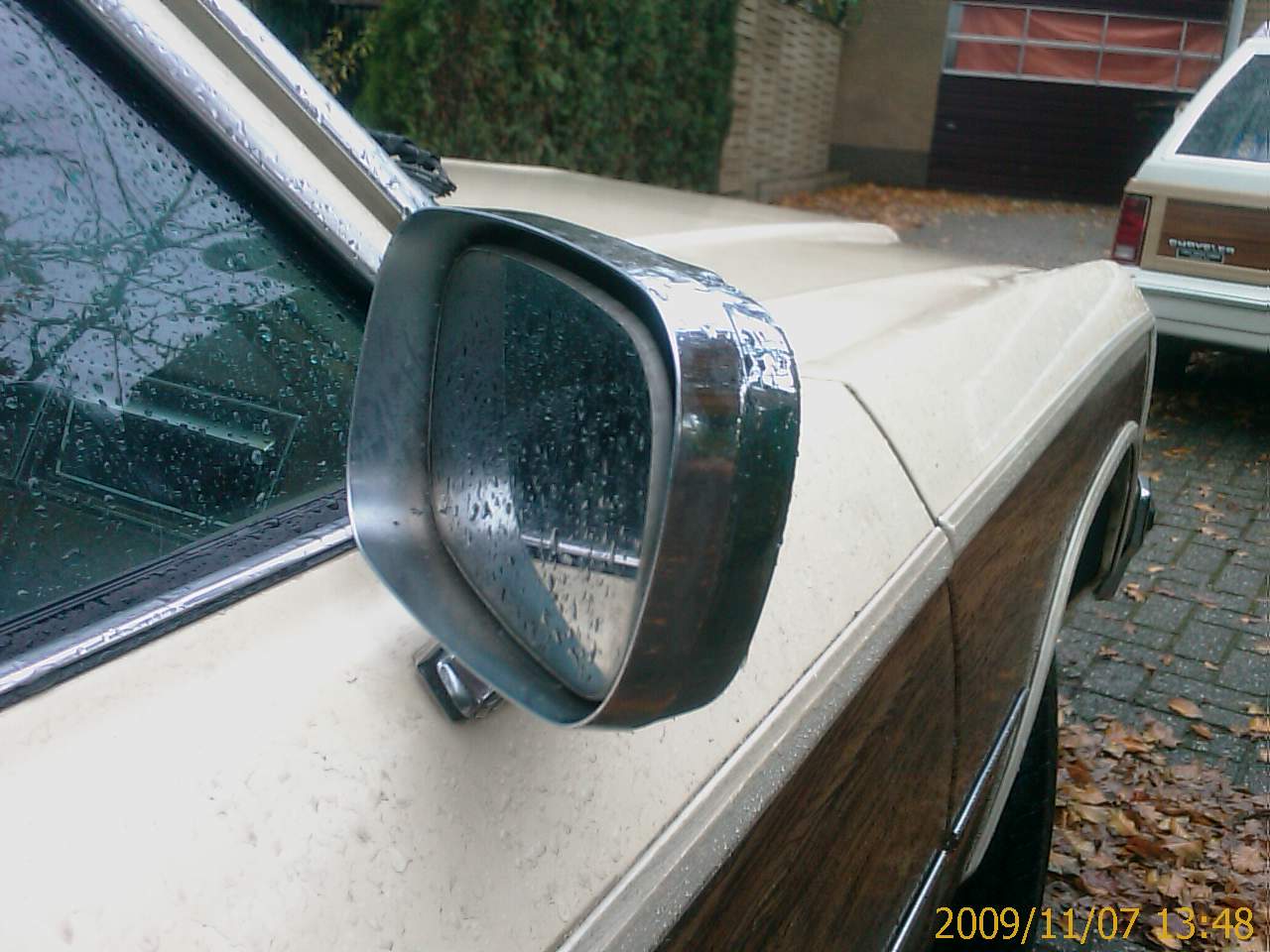A close-up photograph of a classic 80s or 90s Oldsmobile station wagon shows the passenger side, focusing on the chrome side mirror below the square window. The car features a cream-colored upper half and wood grain paneling in the center, with a matching cream stripe along the bottom. A second, identical station wagon is parked in front, visible only by its rear-left corner and tail light. The scene is captured in a driveway paved with gray stones in a square pattern, scattered with a few leaves. In the background, there's a brown garage with windows, partially covered by an orange curtain. On the left, a tan gate and lush greenery frame the driveway. The bottom-right corner of the image displays a timestamp in yellow text: "2009/11/07 13:48." The entire setting appears wet, indicative of light rain.